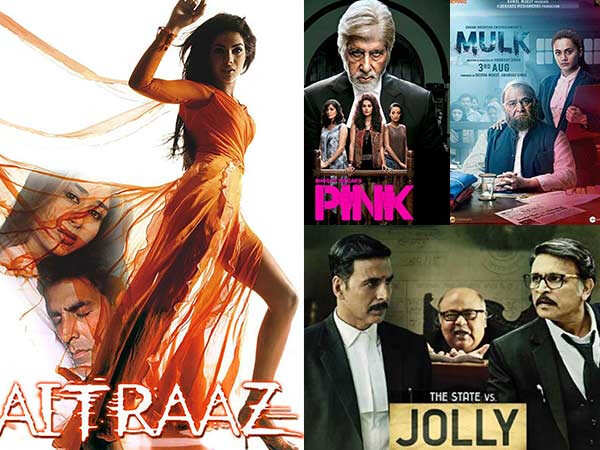The image consists of a main larger panel on the left and three smaller rectangular panels on the right. The left panel, set against a white background, features a woman in a long, gauzy, orange skirt with her legs visible, giving the impression that she is dancing. She has long dark hair and dark eyes, and she appears to be Caucasian. Next to her, a close-up of a man’s and a woman’s faces can be seen, suggesting an embrace. At the bottom, the text "AITRAAZ" is prominently displayed in white letters. The right side of the image is divided into three smaller panels. The top left panel showcases the title "PINK" in pink letters, depicting an older man with three women in front of him. The top right panel displays "MULK" with an incomplete date and features a man sitting at a table with a woman standing behind him. The bottom panel reads "The State vs. Jolly" against a yellow background, showing a judge with two men on either side of him.